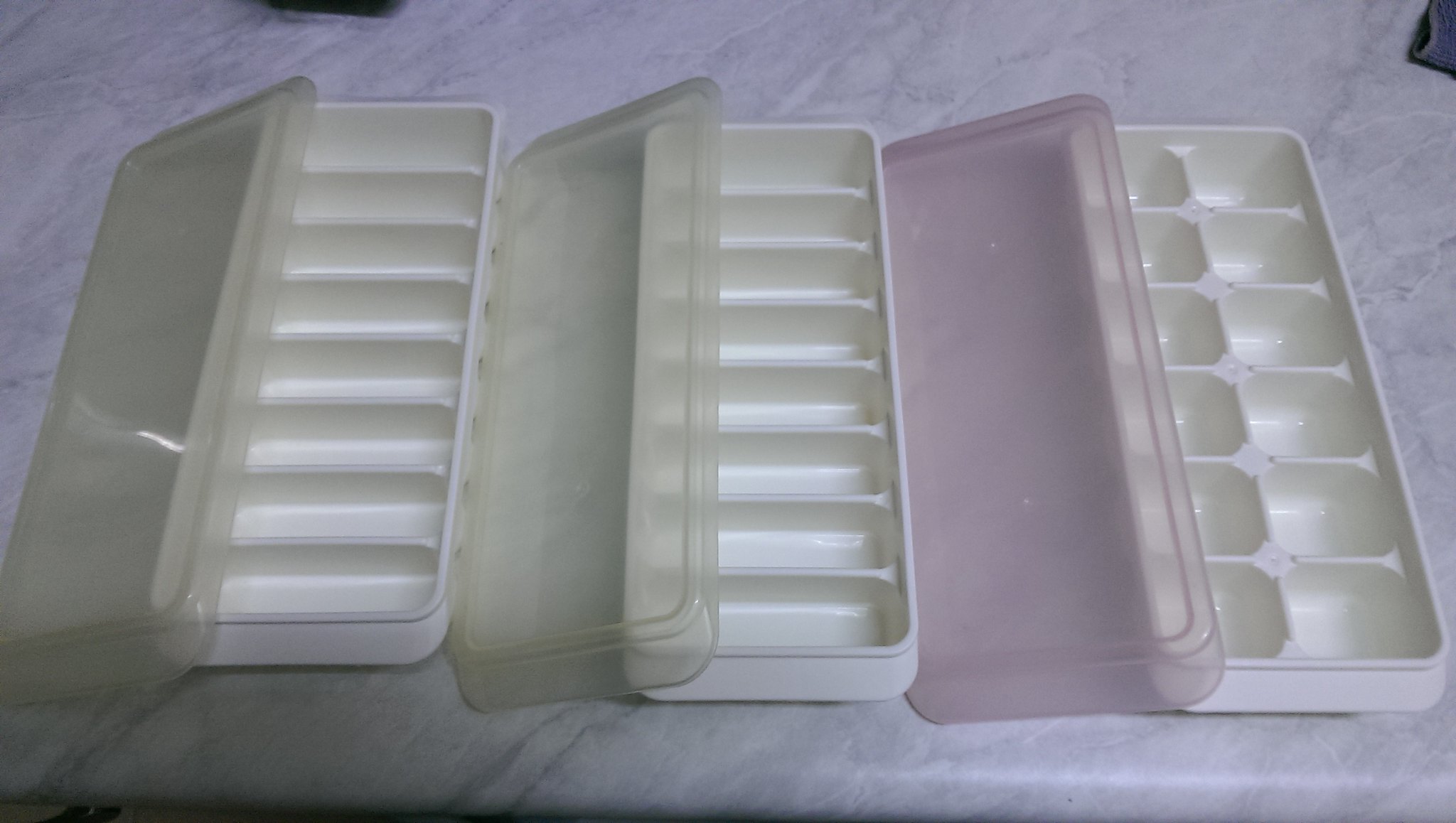The image captures a white marble kitchen countertop with three ice cube trays neatly aligned side by side. The tray on the furthest right is a traditional design with twelve square compartments and a pinkish-hued plastic lid. The two trays to its left feature eight elongated, rectangular slots, each covered with a clear white plastic lid. All three trays share a white base. Additionally, the image has minor details, such as a small gray, folded object in the top right corner and a tiny black sliver in the top left corner, whose identities remain indistinct.